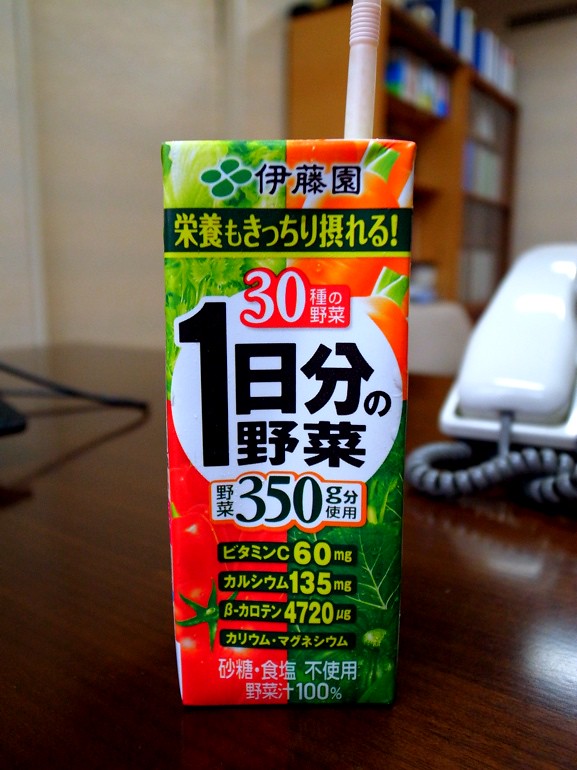The image features a vibrant, colorful cardboard box situated on a wooden table. The box, which seems to contain a beverage or liquid food, is adorned with images of red tomatoes and green cabbage leaves. The label on the box is exclusively in Chinese or Korean script, making it difficult to identify the exact contents. Numerical values are visible on the label, including "30," "350," "60," "135," "4720," and "100%," but their significance is not immediately clear. Positioned at the edge of the table is a white telephone. In the background, there are wooden bookshelves that appear slightly blurred, filled with numerous white books.